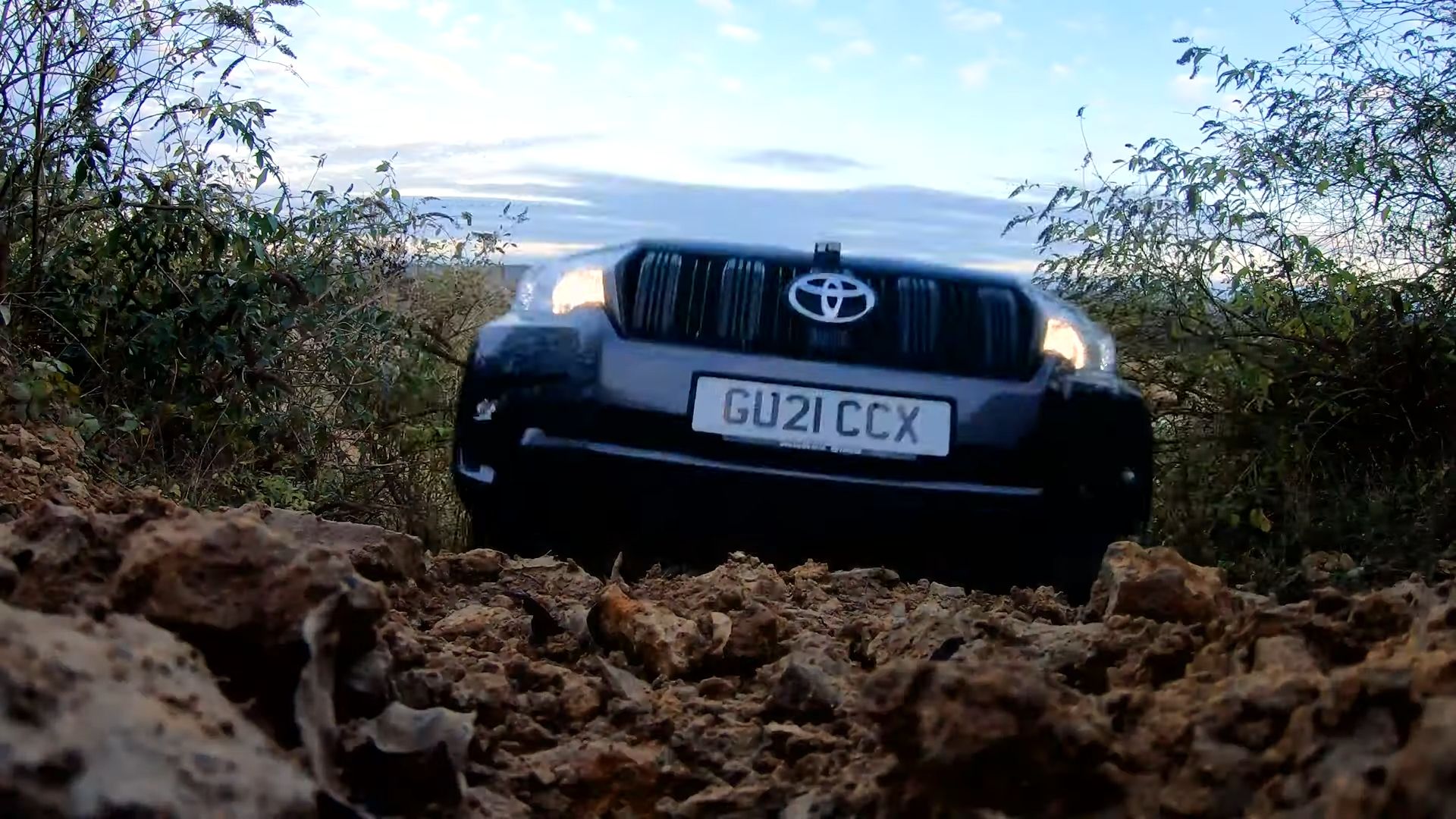The image captures the front of a blue Toyota car, distinct with its emblem centered on the grille and the visible license plate reading GU2ICCX. This is notably a non-American, possibly European plate, distinguished by its larger size compared to the typical U.S. plate. The vehicle is captured driving upwards on a rugged, tan bark-like terrain, filled with jagged rocks, small leaves, and twigs. The photograph, taken from a ground-level perspective looking up, gives prominence to the grille, lights, and bumper of the car, while the rest of the vehicle remains obscured. The vehicle's headlights are on, despite it being a clear daylight scene with a baby blue sky dotted with light clouds. Encircling the car on both sides are vibrant green bushes with long stems and leaves, enhancing the rugged, natural surroundings without touching the car.